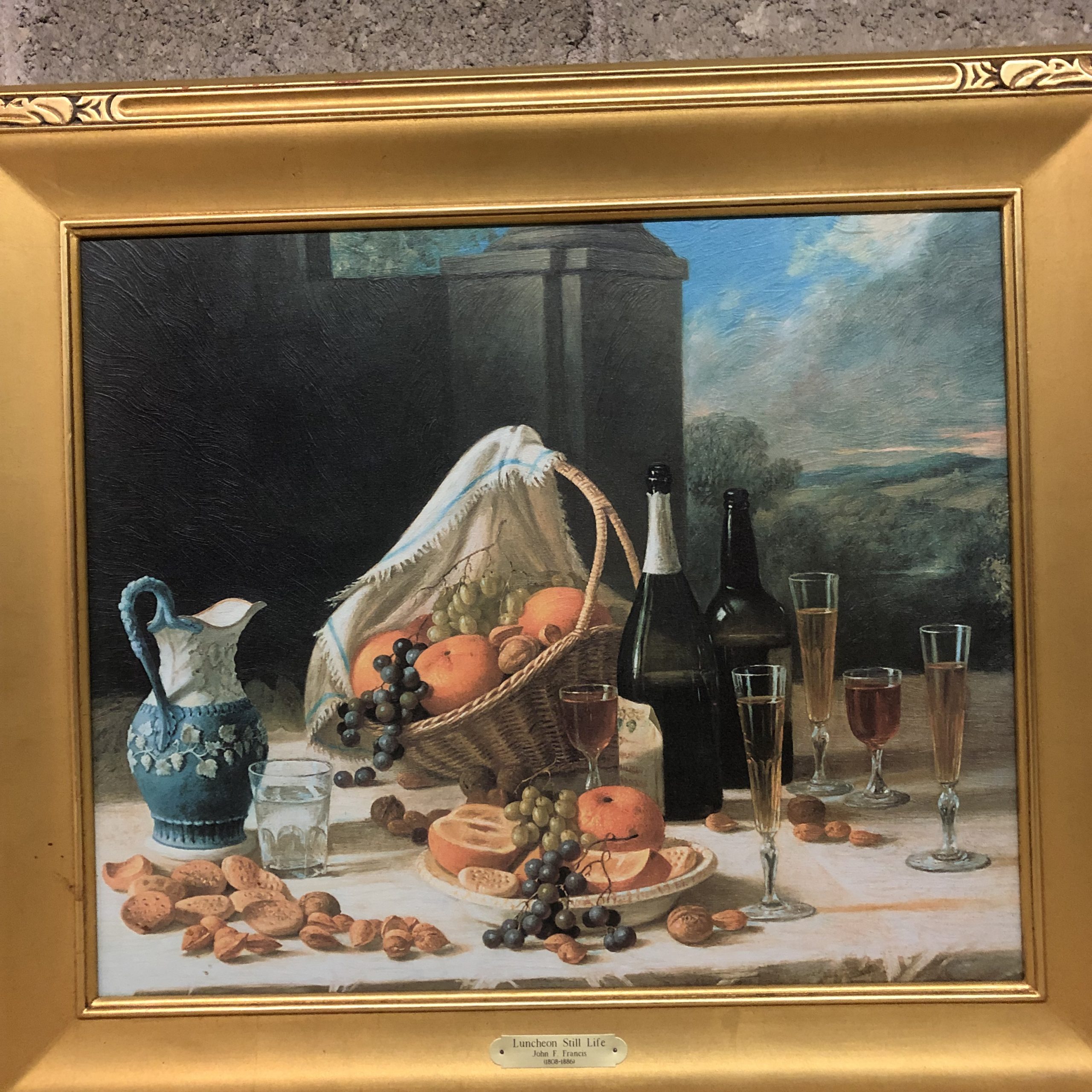This detailed painting, set in an ornate gold frame and titled "Luncheon Still Life" as indicated by a small gold plaque, depicts an elegantly set table on a patio with a scenic countryside backdrop featuring rolling hills, trees, and clouds. The table is draped with a tablecloth and holds a variety of items, including two bottles—one of champagne and one of wine—flanked by three flute glasses and two wine glasses. A large woven basket overflowing with fruits, mainly oranges and grapes, is draped with a dish towel. Scattered across the table are assorted mixed nuts, some yet to be cracked. A white dish also packed with grapes and sliced oranges appears to be brimming to the point of spilling onto the table. Adding to the refined setting, there is a blue and white ceramic pitcher with a leaf pattern, and a pint glass, possibly holding water. The scene's composition, with its detailed elements and background, suggests a luxurious yet leisurely outdoor meal.